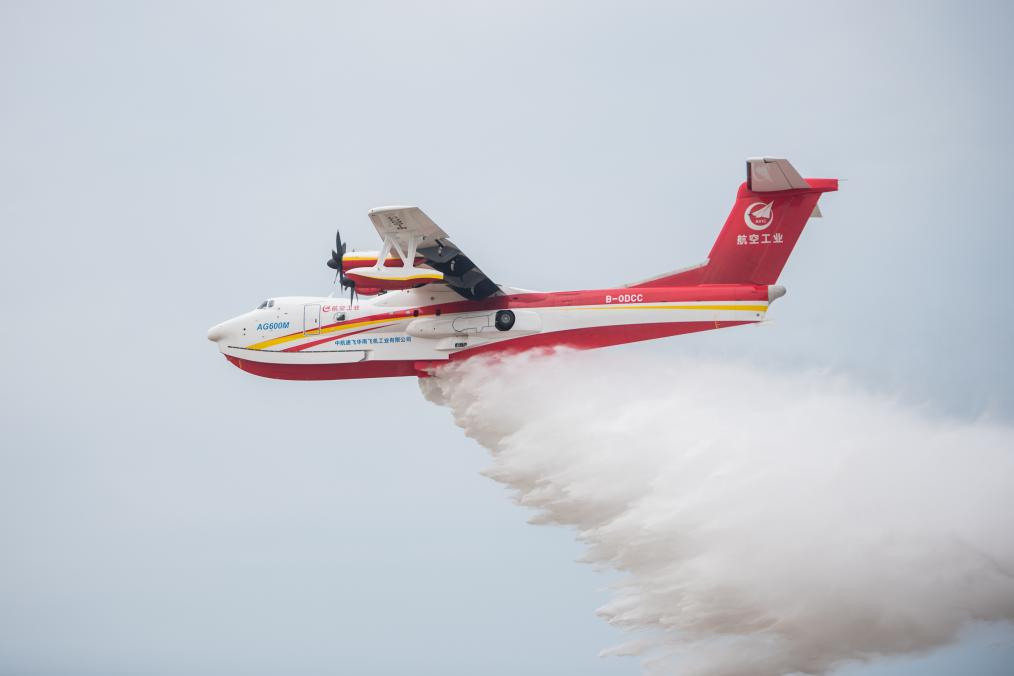In this image, an aerial scene captures a red and white plane flying against a backdrop of dark gray clouds. The airplane has a white nose adorned with a distinctive yellow stripe that transitions into red towards the back. Prominently featured on the side of the plane is the code "B-ODCC". The upper section shows a propeller mounted above the aircraft, contributing to the plane's distinctive design. Additionally, there's blue lettering near the front section which reads "AG-600M". The tail showcases a unique white emblem resembling a paper airplane within a circle, accompanied by Asian lettering. Below the plane, a substantial plume of white smoke trails from the center to the bottom right, suggesting it may be dispersing a substance, possibly pesticides or crop spray. The cockpit faces left, indicating the plane's direction of movement.